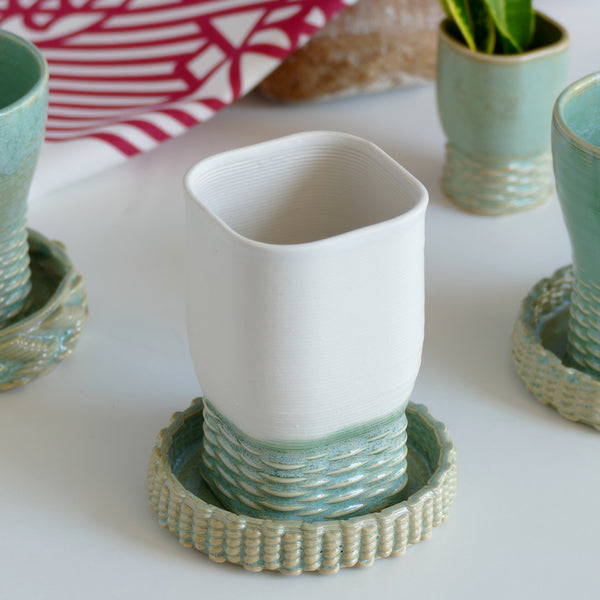The image showcases a cluttered indoor tabletop featuring several small planters, each accompanied by a ceramic saucer. The central planter stands out with its white upper section and pale green base, adorned in a green basket weave pattern. This planter is equipped with a matching saucer and encircled by three similar pots. To its right, two other planters are predominantly green, one hosting tall plant stalks suggestive of a snake plant. There is a partial view of another planter on the left, behind which a white plate with red markings is visible. The planters are neatly spaced, about two to four inches apart, inset from the white tabletop. In the background, a white and red tablecloth and a bag possibly containing soil hint at ongoing or upcoming planting activities.